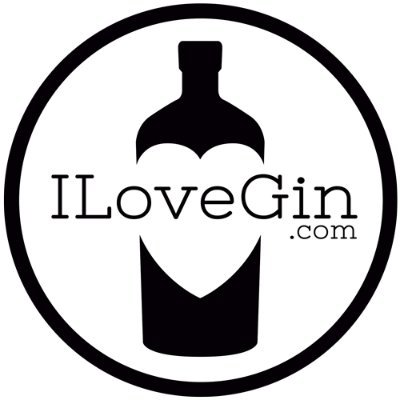The logo is a striking black and white design centered on the text "ILoveGin.com," with the letters I, L, and G capitalized and the rest in lowercase. Positioned below the main text in smaller lettering is "dot com." Surrounding this central text is a black gin bottle that features a prominent white heart shape in its center, which takes up roughly one-third of the image. This heart, created by the white space within the bottle, is centered in the design. Encasing the entire logo is a thick black circular border, completing the sleek, monochromatic appearance.